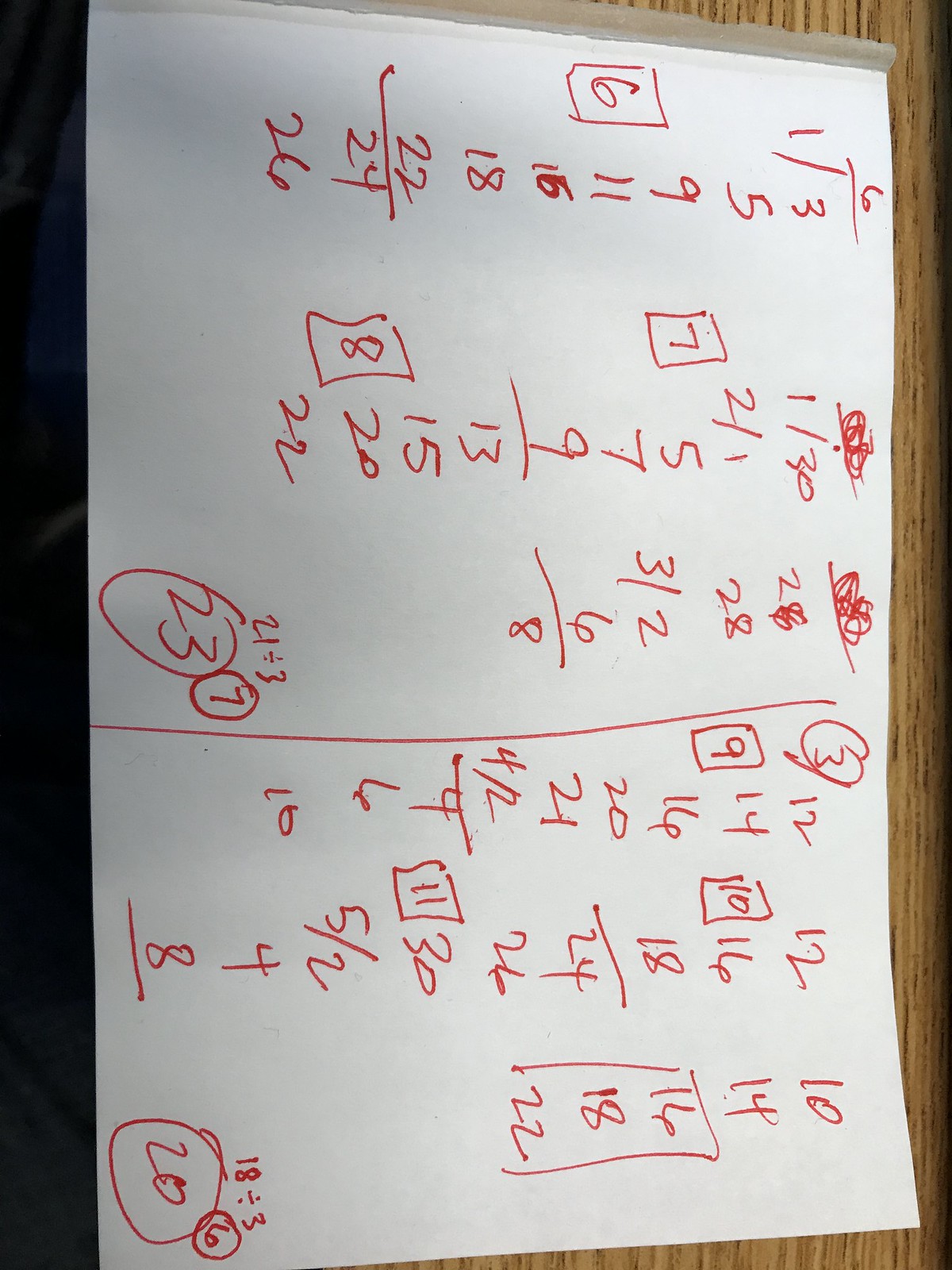A detailed photograph displays a white notepad replete with red numerical calculations, resting on a wooden background. The image is captured in portrait mode but is oriented incorrectly, requiring a tilt of the head to the right for proper viewing.

The notepad, potentially of various dimensions, is filled with intricate mathematical workings. The first column features a fraction 6 over 1/3, followed by the sequence 5, 9, 11. Below these numbers are 6 encased in a box, sequences descending in order as 15, 18, and 22. Below, a line separates the 22 from 24, and 26 is noted underneath, leading to a scratched-out value above another line. Written below that is 1/30, 2, 2 over 1, with successive values of 5, 7, and 9. Another sum line follows, with values 13, 15, 20, and 22 beneath it, accompanied by an 8 in a box to the left of the column. Close by, another scratched-out number is followed by 2 and another scratched-out figure. Descending from these are 28, 3/2, and 6, ending in a sum line marked as 8. Finally, at the column's base are 21 divided by 3, alongside 23 encircled, and 7 in another circle.

To the right, a new segment initiates with a circled 3 beside a 12. Below are values 14, followed by 9 in a square, 16, 20, 21, and 4 over 2, ended by a sum line. Below it are 4, 6, and 10. Adjacent numbers in the neighboring section start with 12, followed by 16, and a boxed 10 underneath. Continuing below are 18, a sum line, 24, 26, and 30. Alongside 30 is 11, boxed, succeeded by 5/2, 4, and 8 beneath a line but no sum below.

In the final column, the sequence starts with 10, followed by 14 in an incomplete rectangle, 16, 18, 22, ending finally with 18 divided by 3. Encircled values at the very bottom include 20 in a circle, and a 6 in a circle.

The extensive content filled with line separations, encased numbers, circled values, and scratched-out elements contribute to a perplexing array of unknown mathematical work.